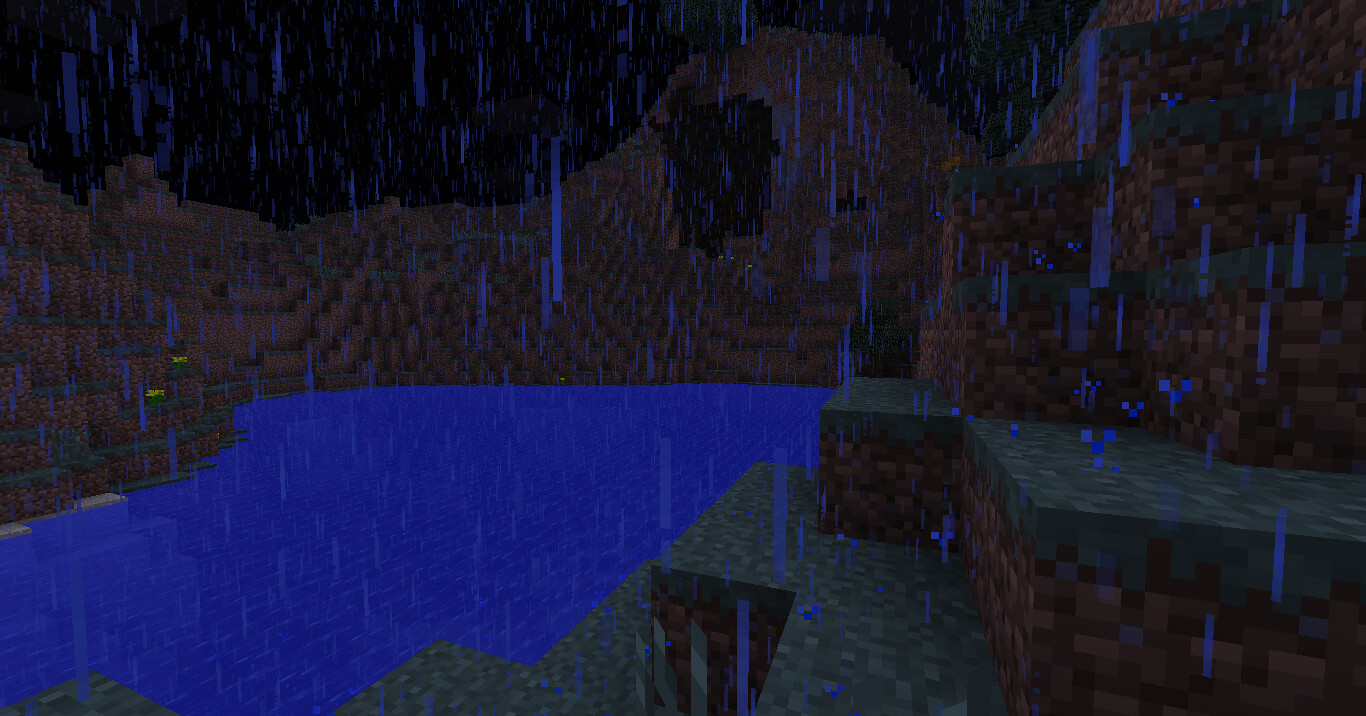This is a detailed screenshot from the video game Minecraft, portraying a nighttime scene under a dark, black sky. In the forefront, rain falls in small, square and rectangular drops, creating a serene yet moody atmosphere. The scene is dominated by a rugged brown cliff that spans across the background from left to right, with a dark cave entrance carved into the middle. Below, there is a small, vivid blue lake nestled at the bottom left of the image. Surrounding the lake, grass blocks are scattered throughout the scene, with some areas of grass and yellow flowers prominently displayed on both sides. The terrain even forms a staircase-like structure on the right-hand side, adding depth and dimension to the landscape. The combination of the falling rain, the night sky, and the natural elements creates a captivating and immersive environment typical of a Minecraft world.